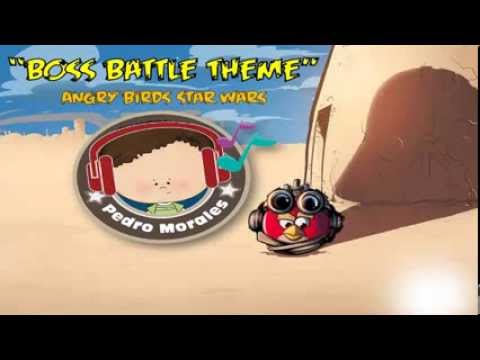In this color illustration resembling a video game still, the landscape-oriented image prominently features a sandy, desert-like setting with a vast beige backdrop. A horizontal black strip runs across both the top and bottom, framing the scene. At the center of the image, there's a brown circle containing a cartoonish, big-headed kid with brown hair and red headphones, identified as Pedro Morales in white text with stars flanking his name. 

To the right is a red Angry Birds character, adorned with steampunk goggles, appearing to emerge from a sandy dune beside a sand hut. The shadow cast by this hut intriguingly mimics the shape of Darth Vader's helmet. Above this central tableau, yellow capitalized letters read "BOSS BATTLE THEME," and below, in golden capitalized letters, it says "ANGRY BIRDS STAR WARS." The overall scene is rendered in a comic book style, blending elements from both the Angry Birds and Star Wars universes.